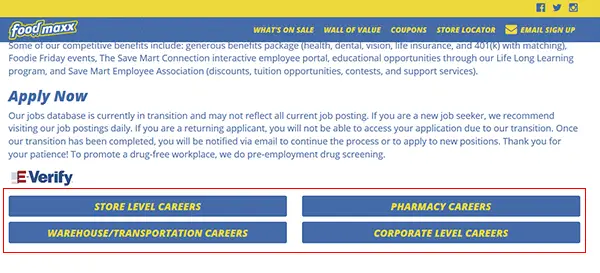In this detailed image of the FoodMax website or app interface, the header bar at the very top is yellow, featuring icons for Facebook, Twitter, and Instagram on the far right. Just below this, there's a blue header bar containing the FoodMax logo on the left, prominently displaying the name "foodmaxx" in lowercase letters with a yellow aura surrounding the text.

Directly beneath the logo is the menu bar with several options: "What's on Sale," "Wall of Value," "Coupons," "Store Locator," and an email signup icon. Below this navigation area, the main content begins with text highlighting the company's competitive benefits, which include generous packages, health, dental, vision, life insurance, and a 401k plan with matching contributions. Additional perks mentioned are Foodie Friday events, the Save Mart Connection Interactive Employee Portal, educational opportunities through their lifelong learning program, the Save Mart Employee Association, discounts, tuition opportunities, contests, and support services.

Following the benefits section, there is an "Apply Now" button, accompanied by directions on how to apply. The image also references E-Verify participation. Career options are presented in a series of blue buttons outlined in red, displayed in a white rectangular box. The store-level careers button is listed first, followed by the Pharmacy Careers button. The next row features buttons for Warehouse/Transportation Careers and Corporate-Level Careers, making it easy for users to navigate their employment opportunities.